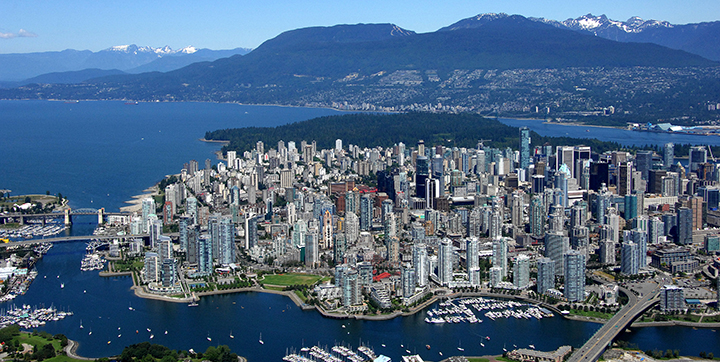The image captures a dynamic and modern cityscape bordered by expansive waterways on three sides, creating a picturesque harbor setting. Overhead, a light blue sky stretches across the top of the frame, providing a serene backdrop to the city. In the distance, imposing mountain ranges rise dramatically, their peaks dusted with white snow, adding to the majesty of the scene. The mountains on the left and right sides possess a bluish hue, while the central peaks are darker, in shades of black or brown, with little to no snow.

The city itself is an impressive display of modern architecture, with numerous tall, silverish skyscrapers that dominate the skyline. The buildings are predominantly white and gray, interspersed with a few brown, black, and blue structures. Below the cityscape, a hillside descends into a densely packed area of smaller houses and buildings, many of which are white and gray as well, blending harmoniously with the tall structures above.

A notable feature of the city is its extensive network of bridges and roads that connect the various sections of the urban landscape. On the left side of the image, a series of bridges span the waterway, while on the right side, a gray road with a yellow line stretches over the water, linking to more land. The shoreline is dotted with white boats, indicating active maritime activity.

In the foreground, there are green trees adding a touch of nature to the urban environment, with some housing areas positioned along the shore. Overall, the image offers a comprehensive and detailed aerial view of a sprawling, water-bound metropolis framed by majestic mountain ranges and connected through a series of elaborate bridges and roads.